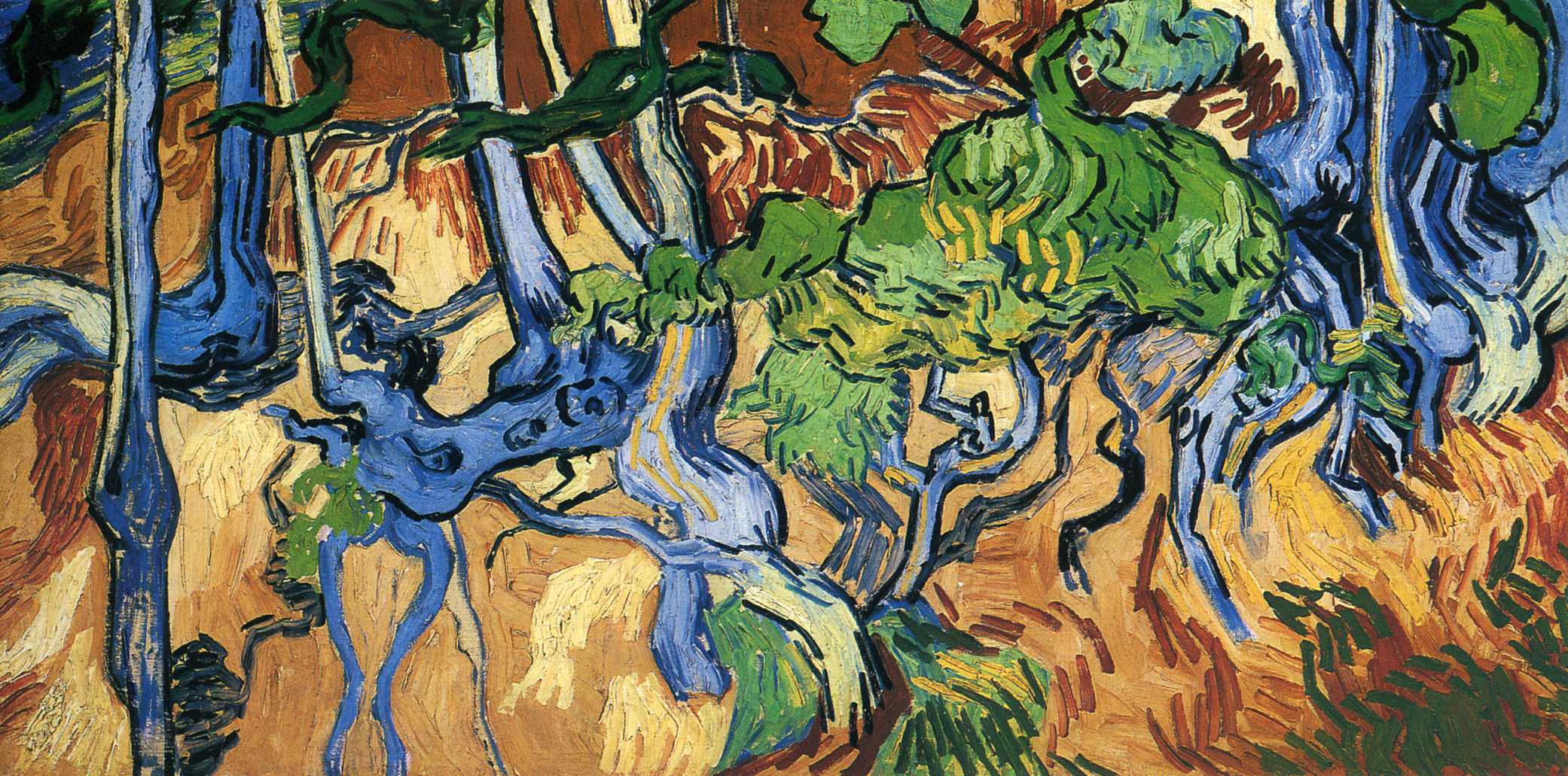This abstract painting is a horizontally aligned, rectangular piece devoid of a border, featuring a vibrant and chaotic interplay of colors and shapes. The background is primarily composed of varying shades of brown, providing a fertile ground-like base. Throughout the painting, there are numerous twisting and swirling elements predominantly in light blue, dark blue, and various shades of green and brown. These serpentine and vine-like forms weave through the composition, sometimes resembling leaves or snakes, and are intricately outlined in black, suggesting a careful and deliberate detailing with pen, pencil, or marker.

The foreground showcases a mix of green, fuzzy figures possibly adorned with yellow, nail-like shapes, which could be interpreted as leaves or other natural appendages. Amidst these, there are blue, elongated, and gnarled branches or stems that stretch across the painting, creating a tangled web of organic forms. These bluish shapes are particularly prominent on the left side, extending vertically and branching out perpendicularly.

Higher up in the painting, patches of vibrant green and yellow punctuate the scene, possibly illustrating vegetation, while large blue feet-like structures, almost humorous in scale, emerge, casting ambiguity on the subject matter. The overall aesthetic evokes a resemblance to Vincent Van Gogh’s brushstroke technique, with long, deliberate strokes of color combining to form an intricate, albeit indiscernible, natural scene. The absence of any text or explicit figures allows the viewer's mind to wander, interpreting the random shapes and vivid colors through their own biases, bringing a wide array of personal interpretations to life.